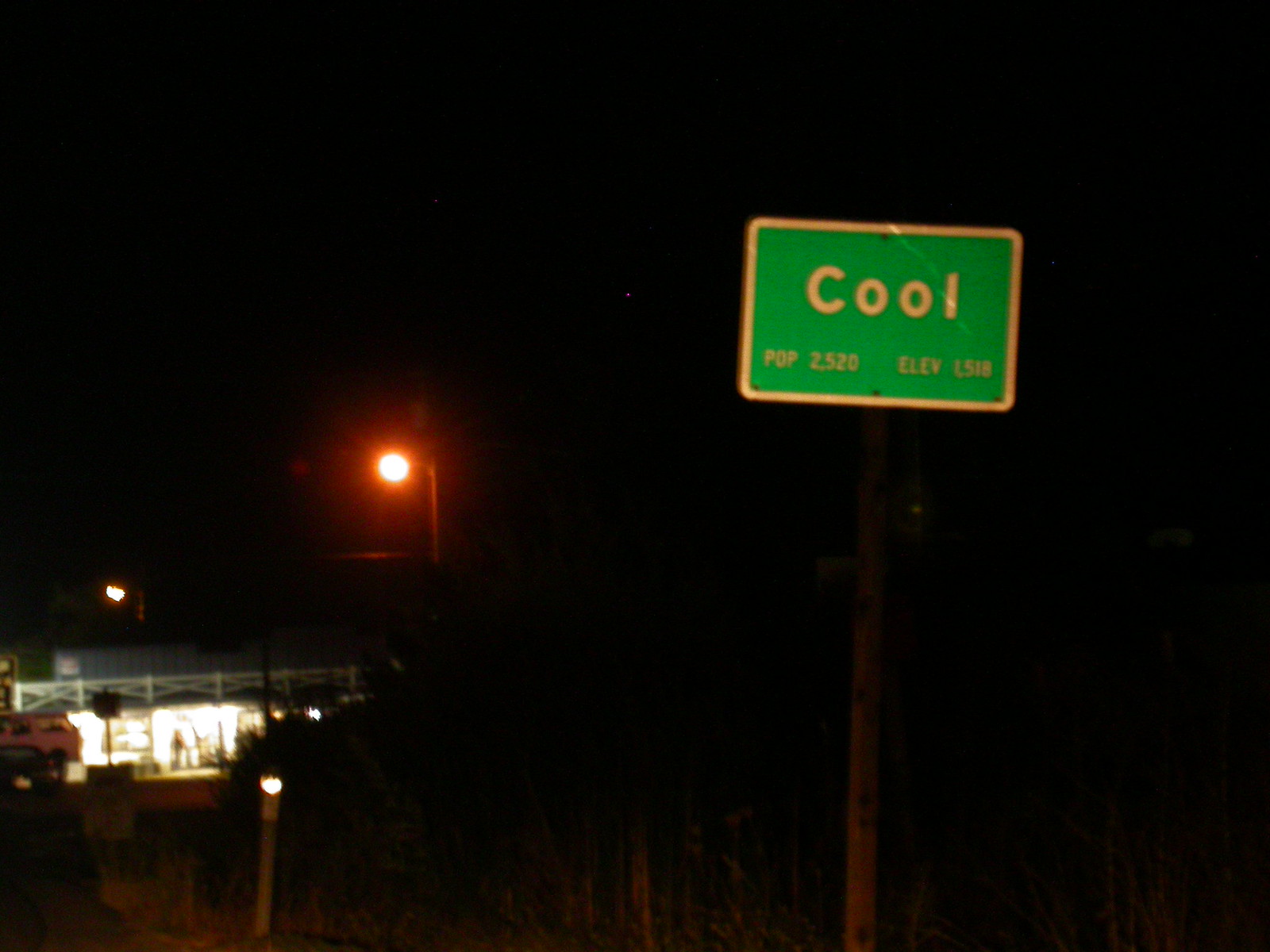In the foreground on the right side of the image, there is a green sign bordered in yellow, prominently displaying the text "PDP 2.522" in violet. To the left of this sign, a structure, possibly a building, can be seen with someone standing inside, illuminated by interior lighting. Adjacent to the building, a pole with an orange light on top stands out. The background and surrounding areas are engulfed in darkness, emphasizing the lit elements in the scene.